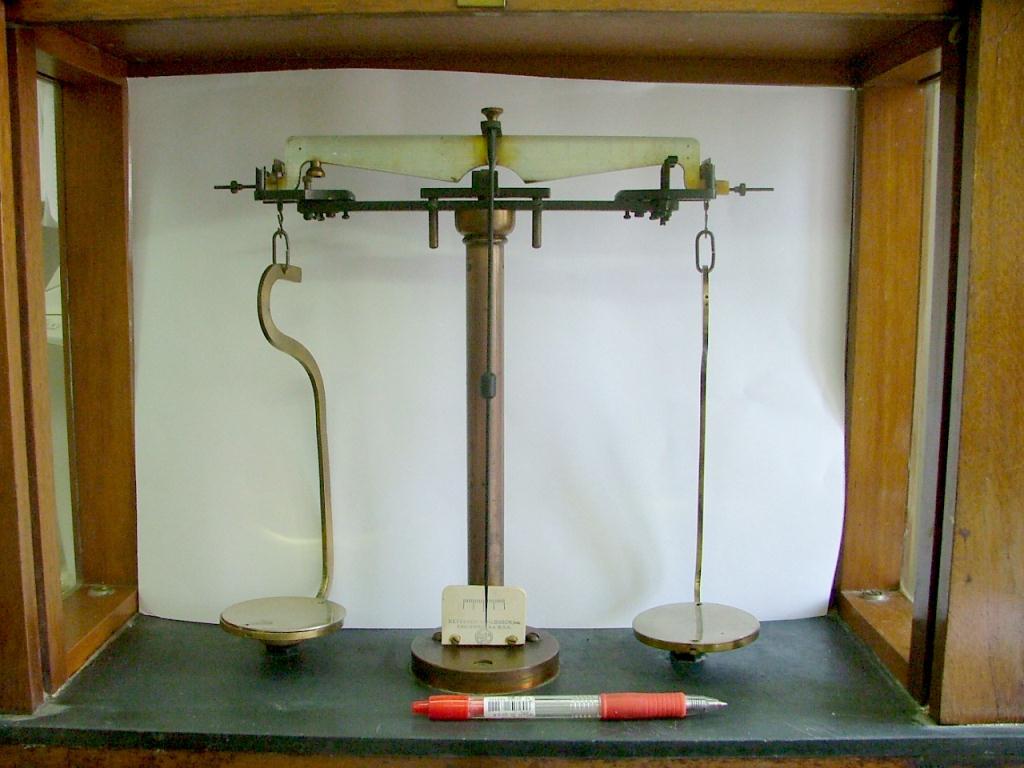This detailed photograph showcases a vintage, old-fashioned mechanical scale device. Positioned on a countertop with a distinct green hue, the scale is framed by a wooden structure, creating an empty space between two wooden pieces. The balance beam of the scale is black, with two gold-colored circular brass discs hanging on each side; the left is thinner with a loop, while the right is thicker and flatter, secured with an S-shaped hook. Central to the setup is a brass pole that holds the balance scales. In front of the scale, there is a striking white and red ink pen, featuring a silver tip and a red thumb grip, placed for size reference. The entire apparatus sits within a setup backed by white paper, adding contrast to the image.